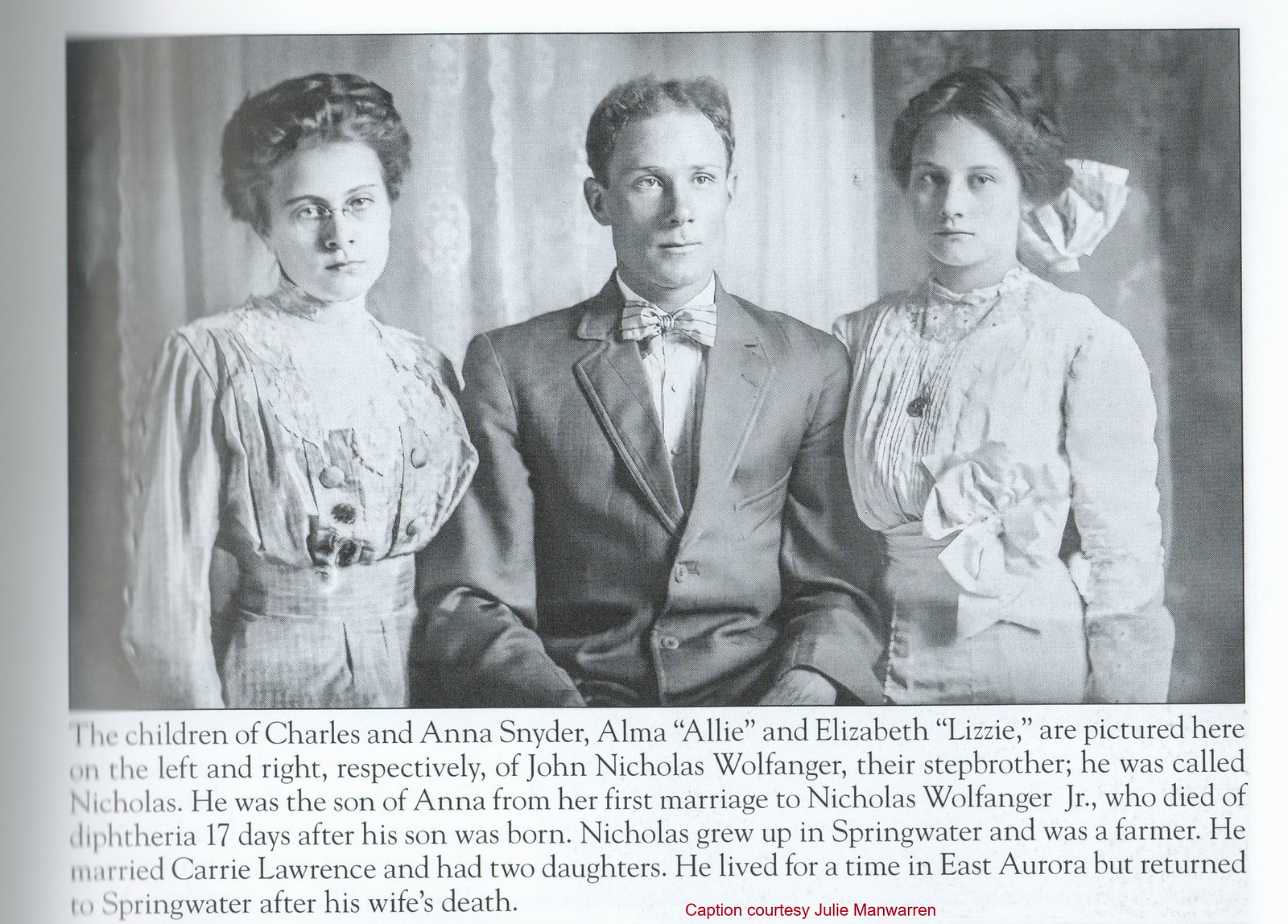This image is a snippet from an old newspaper, featuring a central black-and-white photograph of three well-dressed individuals posed against a curtain backdrop. Sitting in the center is John Nicholas Wolfanger, known as Nicholas, attired in a suit with a jacket, white button-up shirt, and bow tie, his hair neatly parted in the middle and slightly curly. To his left stands Alma Snyder, adorned in an ornate dress that cinches at the waist and billows at the stomach and sleeves. Her hair is styled in a brain-like pattern and she wears thin wire glasses. To his right is Elizabeth Lizzie Snyder, appearing younger, with her hair pulled back and accented by a large white ribbon. She is dressed in a similar white, poofy dress and wears a locket. Below the photograph, the text explains, "The children of Charles and Anna Snyder, Alma, Allie, and Elizabeth Lizzie, are pictured here on the left and right, respectively, of their stepbrother, John Nicholas Wolfanger." Nicholas was the son of Anna from her first marriage to Nicholas Wolfanger Jr., who died of diphtheria 17 days after his son was born. Nicholas grew up in Springwater, became a farmer, married Carrie Lawrence with whom he had two daughters, and later returned to Springwater after living in East Aurora following his wife's death. The photograph’s style and accompanying text echo the aesthetic and narrative style typical of historical newspaper features.